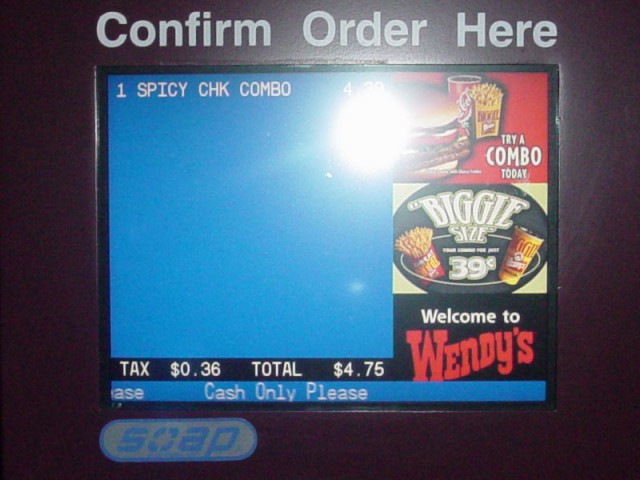The image depicts an old interface on a Wendy's fast-food restaurant order screen, possibly at a drive-thru. The top of the screen features the text "Confirm Order Here" in white. Below this, on the left side, is a light blue background displaying the order "One Spicy CHK Combo - $4.39" in white text. A bright white light obscures part of the price. To the right, a red square showcases a hamburger, a cup of Coke, and some french fries, urging customers to "Try a Combo Today." Just below it, another box advertises "Biggie Size 39 cents" with images of fries and a yellow cup. Further down, a black square displays “Welcome to Wendy's,” with "Welcome" in white and "Wendy's" in red. The bottom of the screen details the tax (36 cents) and the total ($4.75). A blue bar underneath reads "Cash Only Please," and at the very bottom is an oval with a blue outline and a gray background containing the text "SOAP."